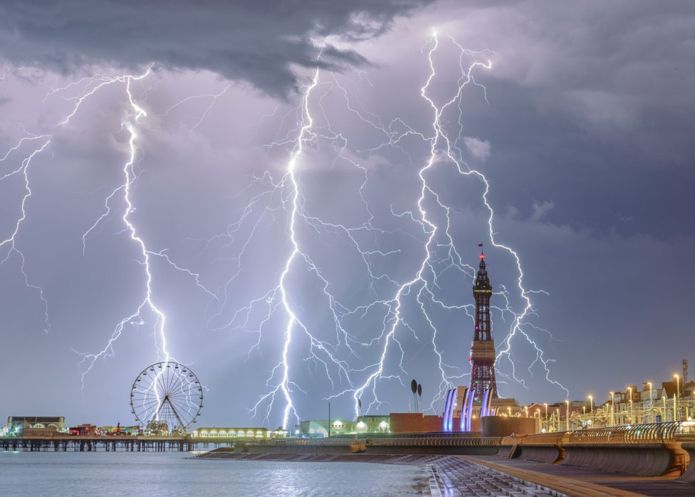In this striking image captured during a lightning storm in the early evening, the scene unfolds over a bustling waterfront area dominated by a pier extending to the left. A vibrant Ferris wheel commands attention on the pier, seemingly silhouetted against the stormy backdrop. Four vivid bolts of lightning streak down from the heavily clouded sky, with tendrils branching out dramatically. One lightning bolt dramatically pierces the sky behind the Ferris wheel, while others strike various points—the pier, the cityscape, and a solitary, tall tower that stands prominently to the right. The foreground features a dark, tumultuous ocean concentrated in the lower left. The city to the right is aglow with numerous streetlights, adding a stark contrast to the stormy, dark gray skies above. Despite the chaotic weather, the scene is alive with electrifying beauty, the brilliant lightning revealing the silhouettes of otherwise distant and indistinct landmarks.